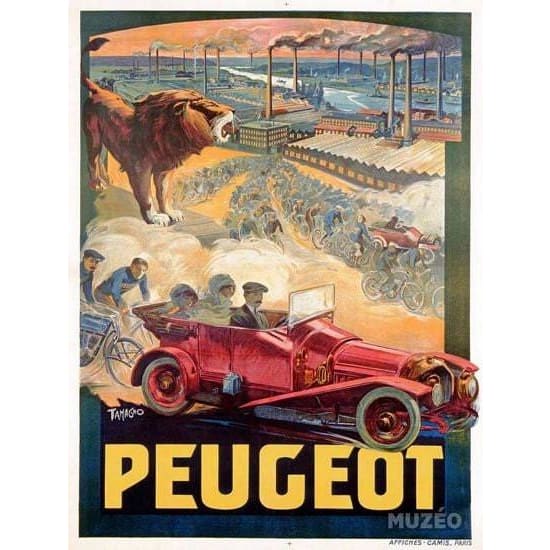The image is a detailed and captivating retro-style poster, likely an advertisement for an old car brand named "Pugiot." Dominating the top left of the drawing is a roaring brown lion perched on a hill, adding a dramatic flair to the scene. The background features a setting sun that bathes the sky in warm orange hues, contrasting with the industrial landscape filled with smokestacks and factories emitting gray smoke. A striking red convertible car with three people seated in it is prominently positioned in the foreground, drawing immediate attention. Behind the red car, two individuals ride bicycles, while a stream of people on motorcycles or bicycles, alongside other vehicles, emerges from the factory. Clouds of dust swirl around these activities, portraying a sense of movement and commotion. The bottom of the poster features bold yellow capital letters spelling "PUGIOT," and just above this is the word "Tamago." The bottom right corner bears the name "Museo" against a blue background, possibly indicating a museum or exhibition element related to the poster.